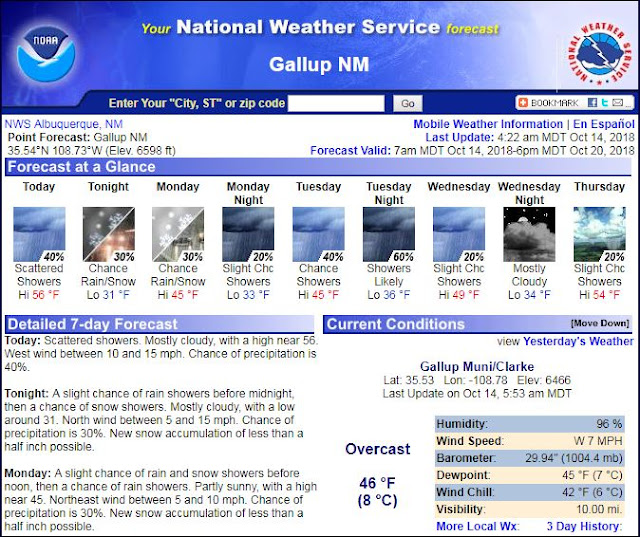The image depicts a web page from the National Weather Service forecast. At the very top, there is a prominent logo on both the left and right sides, representing the National Weather Service. Centrally located is a text field prompting users to enter their city, street, or zip code for a localized weather forecast.

The forecast section is titled "Forecast at a Glance" and provides detailed weather updates:
- Today: Humidity at 40%, with a 40% chance of scattered showers.
- Tonight: Humidity drops to 30%, with a 30% chance of rain or snow.
- Monday: A 30% chance of rain or snow continues.
- Monday 9th: A reduced 20% slight chance of showers.
- Tuesday: A 40% chance of showers.
- Tuesday 9th: An increased 60% likelihood of showers.
- Wednesday: A 20% slight chance of showers during the day, transitioning to mostly cloudy conditions by the evening.
- Thursday: A 20% slight chance of showers.

This detailed forecast layout allows users to anticipate weather conditions with precise percentage chances, helping them plan their activities accordingly.